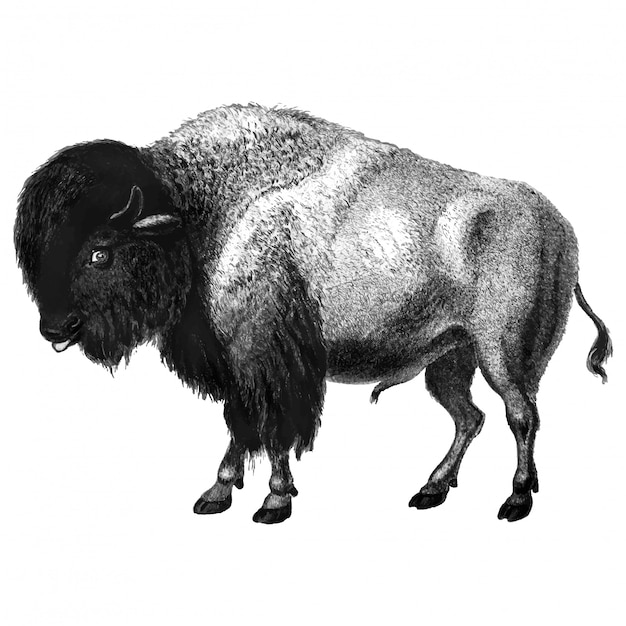This black-and-white artwork appears to be a pencil drawing of a bison standing against a completely white background. The bison, possibly a young adult, is oriented to the left side of the image. Its head is densely covered in a rich, black, fluffy fur, extending into the neck and chest areas, and it possesses large, bright eyes that stand out. The fur lightens into various shades of gray as it continues down the body, transitioning to a lighter hue towards the hindquarters. The bison’s front legs are dark and merge into black at the hooves, while its hind legs appear somewhat lighter due to less fur coverage. The tail is short, ending in a tuft of black hair. The detailed pencil strokes capture the texture and layering of the bison's fur, illustrating contrasts from the very dark head to the lighter back, studded with darker specks.